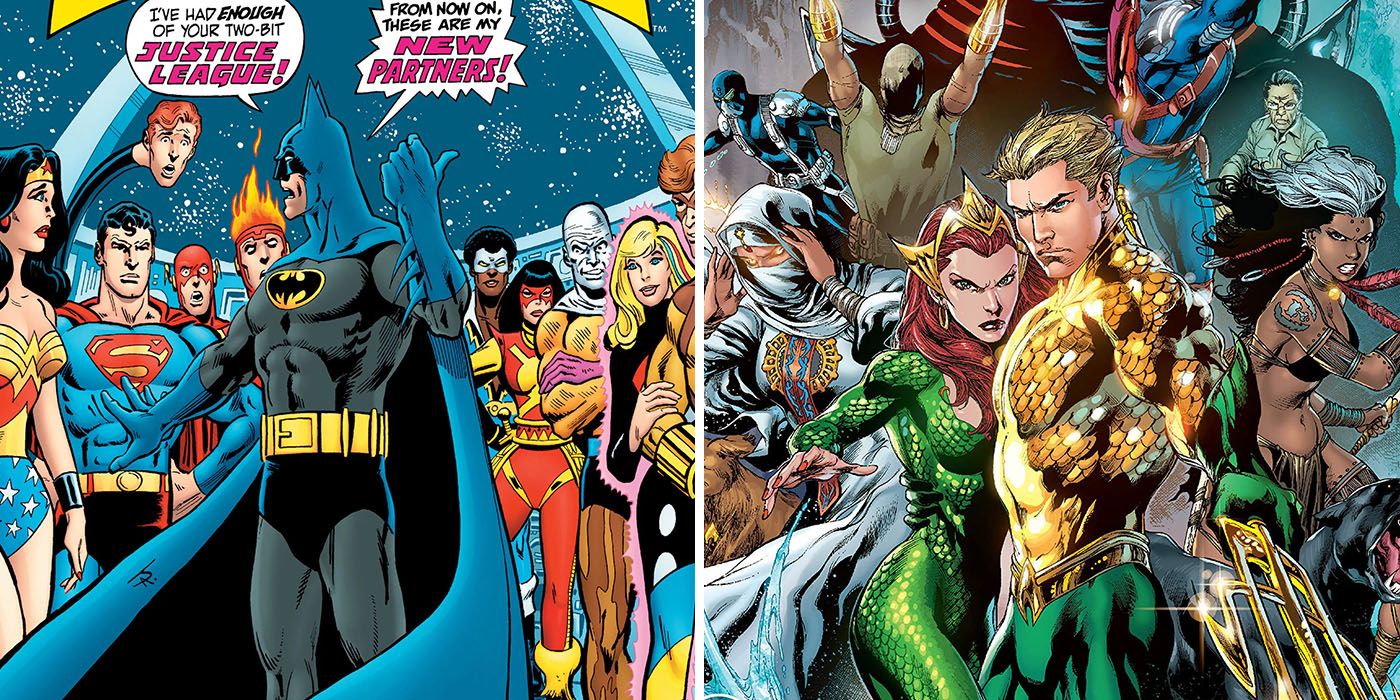In an intense two-panel comic strip from DC Comics, Batman stands at the forefront of a confrontation, clearly taking charge. In the left panel, he wears a gray skintight suit with a blue cowl, cape, and gloves. His left hand is raised with a thumb slightly out, expressing determination while he glares left with his mouth slightly open. Around him, Wonder Woman looks worried, Superman appears angry, and The Flash seems shocked; various other heroes also react to his words. Batman's dialogue in white text bubbles reads, "I've had enough of your two-bit Justice League," with "Justice League" highlighted in pink, followed by a jagged bubble stating, "From now on, these are my new partners," with "new partners" in pink text.

The right panel shifts focus to Batman's proclaimed new allies, led by Aquaman and his forceful-looking partner. Aquaman stands wearing a gold scaled skintight outfit and a green glove, holding a golden trident. His short blonde hair is swept back as he glares ahead angrily. Beside him, his partner dons a scaly green outfit, a gold crown, and has intense bright red hair. Various other distinctive heroes, some shrouded and others more identifiable, align behind them in dynamic poses, ready for action.